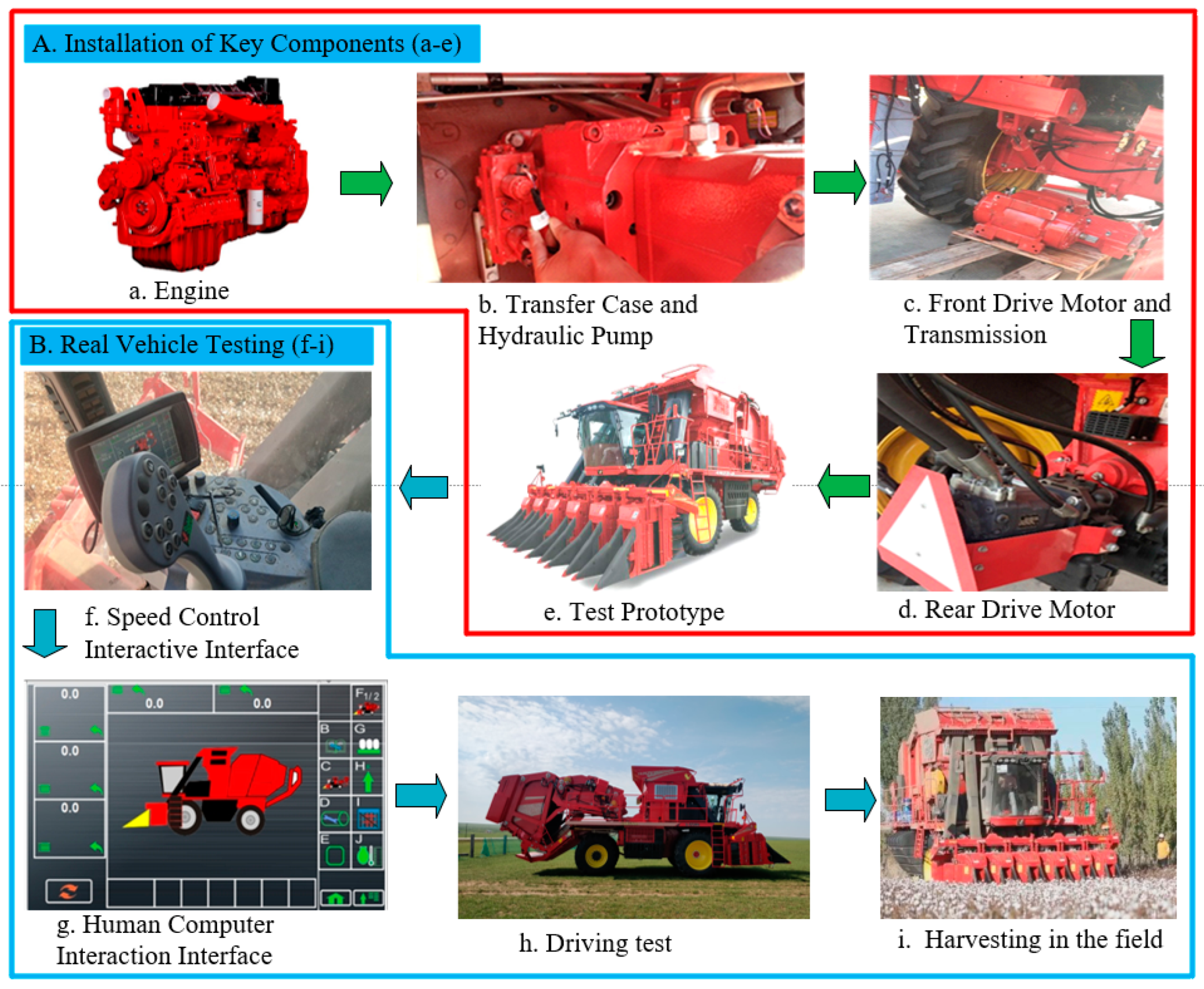The image is a detailed diagram of a red mechanical harvester primarily used for farming. This comprehensive visual guide is segmented into nine distinct images, encapsulated by red and blue polygons—the red on top and blue on the bottom—to differentiate between stages of assembly and operational testing. The sequence begins with a schematic labeled "A," showcasing the red engine followed by "B," highlighting the installation of the transfer case and hydraulic pump. "C" illustrates the front drive motor and transmission, leading to "D," which depicts the rear drive motor. The test prototype phase, marked as "E," concludes the assembly section.

Transitioning to the operational aspects enclosed within the blue polygon, "F" demonstrates the speed control interactive interface, followed by "G," the human-computer interaction interface with an LED screen likely displaying vital metrics like RPMs. "H" shows a driving test image from within the cab, and the sequence concludes with "I," representing the harvester actively harvesting corn in the field. This diagram, which could function well as a poster in a tractor showroom, provides a meticulous breakdown of both the construction and use of this agricultural machine, making it a valuable resource for understanding its mechanics and operation.